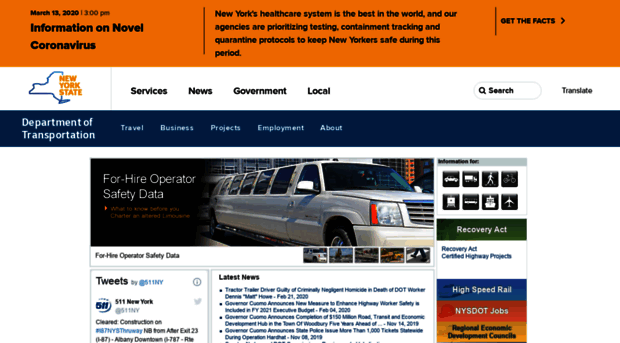The image showcases the homepage of the New York State Department of Transportation website. At the very top, an orange banner is prominently displayed, featuring a special pop-up notice related to pandemic information concerning the novel coronavirus, including a specific date and an important announcement. Below the banner, the main section of the website displays a blue outlined map of New York State with yellow text labeling it as "New York State." This segment also includes various clickable links like Services, News, Government, and Local, situated beneath the state logos.

On the right side of this section, there is a search bar and a translate button for user convenience. A teal-colored bar runs horizontally across the website, bearing the text "Department of Transportation," with smaller writing below it that begins with "Travel" and continues as a resource title, which is partially obscured. Additionally, a black text box contains the phrase "For Hire Operator Safety Data," accompanied by an image of a white stretch limousine.

The website also integrates a social media feed displaying the latest news tweets from the department, along with several thumbnail photos for additional updates and news links. Several interactive icons are available for clicking, including those for directions, airplane travel, and walking, organized into two rows of four icons each below the section marked "Recovery Act." Overall, the website design features numerous small, detailed elements for comprehensive user navigation.